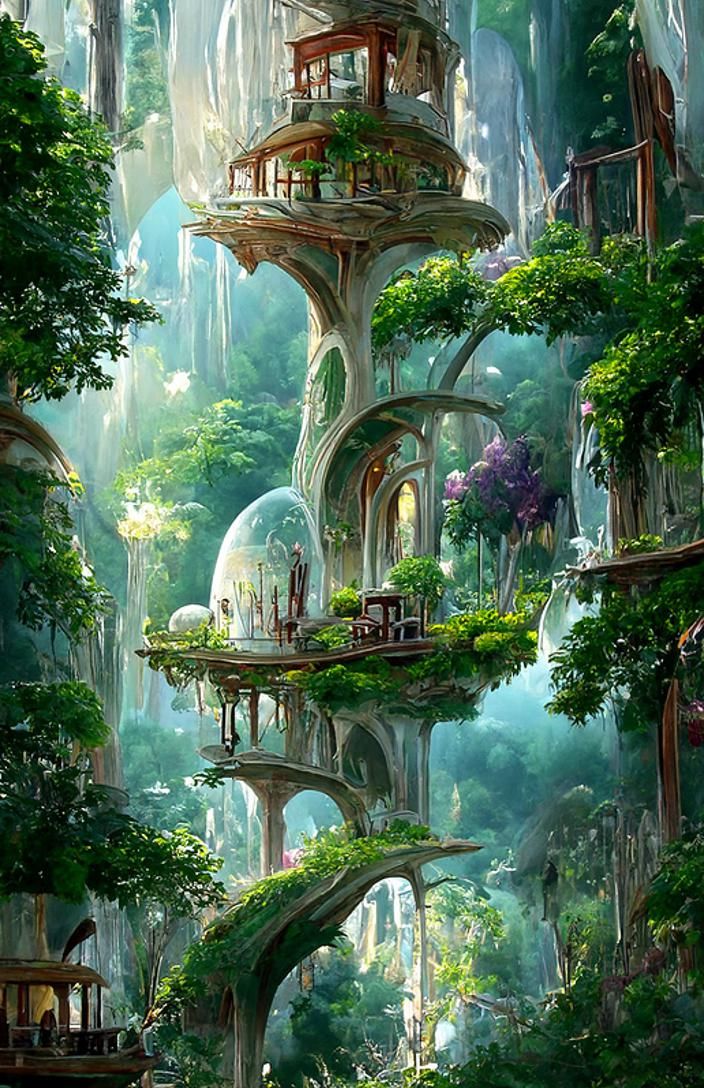The digital fantasy painting depicts a lush, green solar punk setting—a deep forest with a sprawling, multi-leveled, treehouse-like village. Central to the artwork is a tall, grayish-white tree trunk structure, detailed with various levels of living spaces, each encased in glass and adorned with greenery. At the top, there are roofed home fixtures containing cozy bedrooms and visible furniture. Below, glass-encased rooms are furnished with chairs, tables, and other adornments. Branches and plant life are integrated throughout the structure, adding to the naturalistic ambiance. In the bottom left corner, another wooden home is nested within the verdant surroundings, and distant waterfalls cascade through the dense jungle foliage, contributing to the colorful and vibrant scene. The image captures a harmonious blend of nature and dwelling, encapsulating the essence of a surrealist, solar punk utopia.